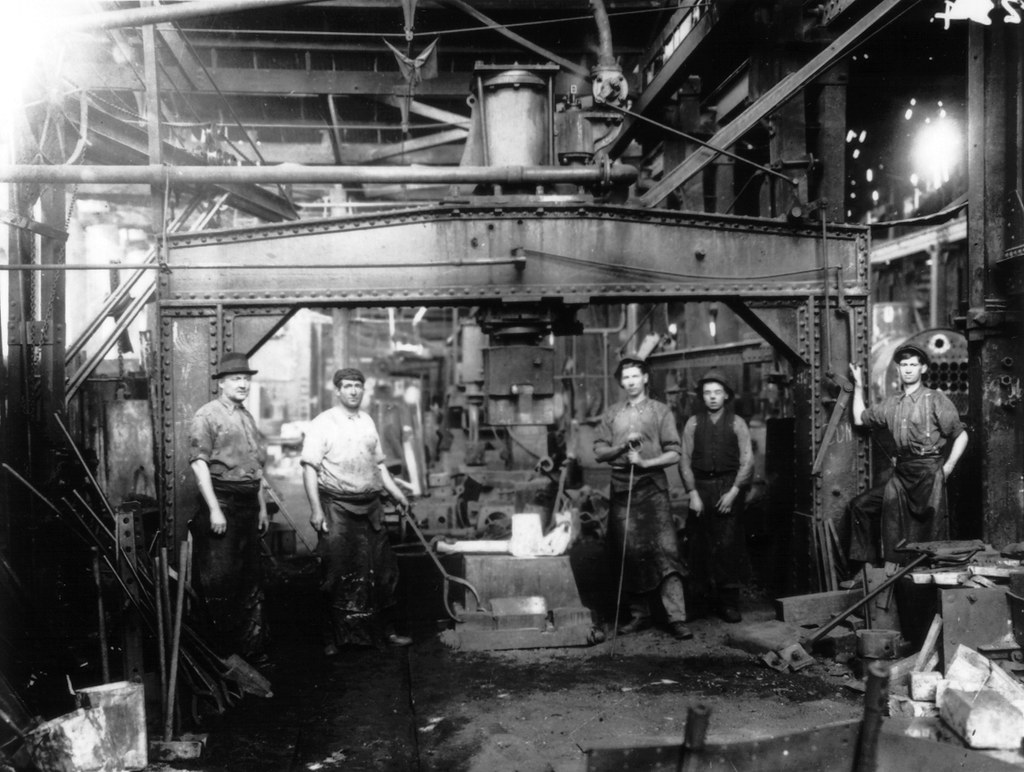In this evocative black-and-white photograph, captured possibly in the 1950s, five men stand in a dark, industrial environment that recalls the gritty atmosphere of a machine shop or potentially a steel mill. The setting is crowded with metal pieces, pipes, and heavy machinery, indicating the demanding, labor-intensive nature of their work. An overhead steel beam spans the scene, reinforcing the industrial atmosphere. The men are lined up horizontally, staring directly at the camera, suggesting they were aware of the moment being documented. To the far left, a man dons a hat; next to him, a man with rolled-up sleeves wears a white shirt. The middle figure grips a large pole, while the man to his right sports a sweater vest. The person furthest on the right is clad in overalls, his right hand resting on the steel beam. A light source at the top right of the photo, possibly sunlight or an artificial light, illuminates the scene faintly from a nearby window. This photograph encapsulates the essence of manual labor during a bygone era, capturing both the camaraderie and the harsh conditions faced by these industrious men.